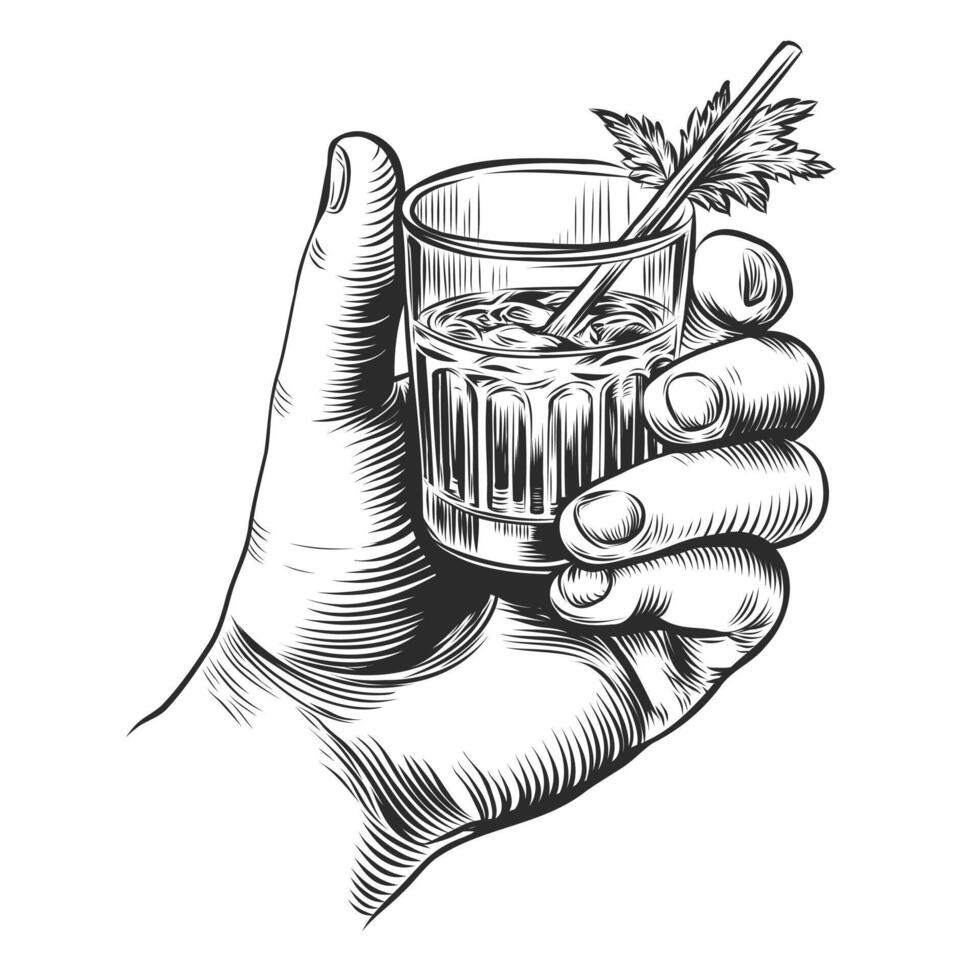This is a highly detailed black and white digital drawing, mimicking a pencil or pen and ink style, depicting a male hand holding a glass. The hand, originating from the bottom left corner of the image, features detailed texturing and shading, with thick black lines highlighting the palm and small fingernails visible on the fingers. The glass, appearing to be clear and plastic, is grasped securely by the fingers and is about three-quarters full of an unspecified liquid. Emanating from the glass is a straw, leaning towards the right, and a decorative sprig with jagged leaves pointing in multiple directions—left, up, and right. The background remains completely white, drawing focus solely to the meticulously rendered hand and glass. This intricate illustration captures the simplicity and potential elegance of what could be a cocktail, possibly a mint julep, accentuating the detailed line work around the hand and glass.